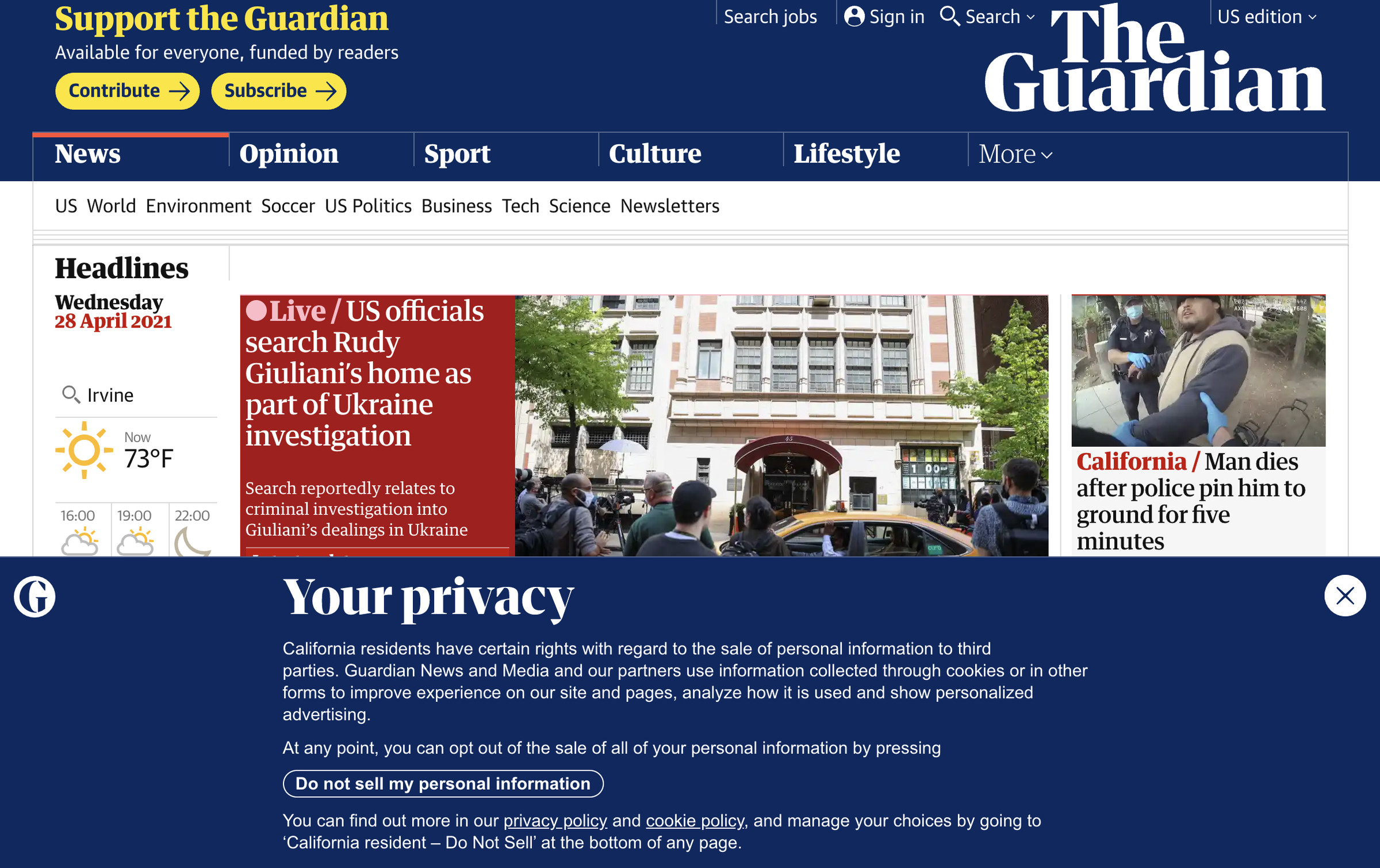The Guardian's website features a predominantly dark blue background. In the upper left corner, there is a yellow banner that reads "Support The Guardian." Positioned beneath it, in white text, are the words: "Available for everyone, funded by readers." Adjacent to this text are two yellow buttons—one labeled "Contribute" with a right arrow, and the other labeled "Subscribe" with a right arrow.

On the upper right side of the webpage, the text reads "Search job," "Sign in," and "Search" with a drop-down menu. The Guardian's logo appears in large white font, followed by "US Edition" also in white, accompanied by a drop-down menu. Directly beneath this header, there is a navigation bar listing categories such as "News," "Opinions," "Sports," "Culture," "Lifestyle," and "More," the latter with a drop-down menu. The "News" section is highlighted with a red line above it, indicating the current selection. Sub-categories under "News" include "US," "World," "Environment," "Soccer," "US politics," "Business," "Tech," "Science," and "Newsletters."

The main content area features the headline for Wednesday, April 28, 2021, which states: "Live US officials search Rudy Giuliani's home as part of Ukraine investigation; search report relates to criminal investigation into Giuliani's dealings in Ukraine."

Additionally, a large banner appears below the main content area, featuring the bold white text "Your Privacy," informing California residents of their rights concerning the sale of personal information to third parties by Guardian News and Media and their partners.